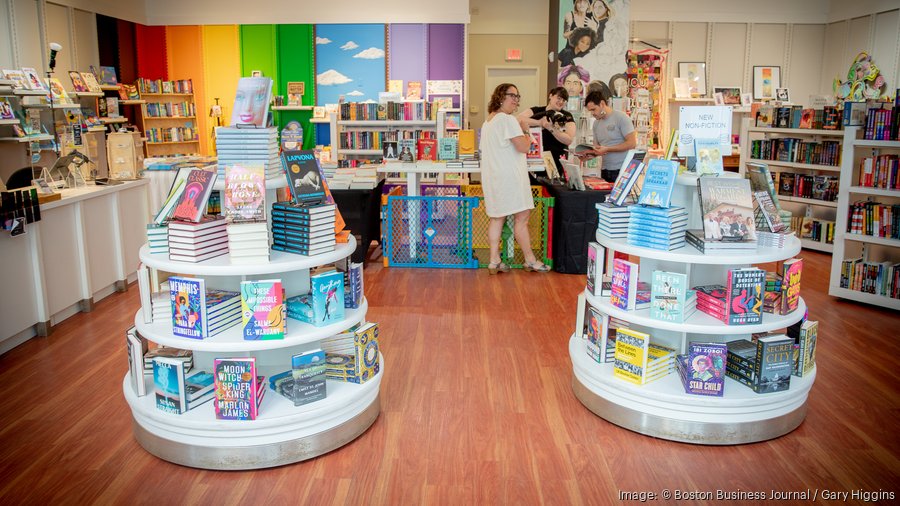The indoor daylight photograph of a vibrant bookstore features white walls with a striking rainbow mural on the back left wall. This colorful display transitions from black to dark red, red, orange, yellow, light green, green, light blue with clouds, to light and dark purple. The store's brown hardwood floors create a warm ambiance, dotted with various white book shelves packed with an array of colorful books in conventional arrangements and decorative displays.

Central to the scene, two large, three-tiered round white book displays stand on either side of center, resembling multi-layered cake platforms, brimming with books arranged both vertically and horizontally. A counter at the back wall hosts a black-shirted employee holding a small black and white puppy. The employee's attention appears divided between the pet and assisting customers.

Three primary customers populate the scene. To the left of the employee, a woman in a knee-length white dress and green heels stands gazing inquisitively, her brown shoulder-length hair complemented by black glasses. To the right, a fit man with short black hair, clad in a gray t-shirt and obscured pants, examines an open book. A back area with an exit sign and a fenced section suggest possible designated spaces within the shop, adding layers of spatial organization.

The foreground and background details culminate in a vibrant yet cozy atmosphere, punctuated by the interaction of people and the colorful spectrum captured in the store's inviting layout.